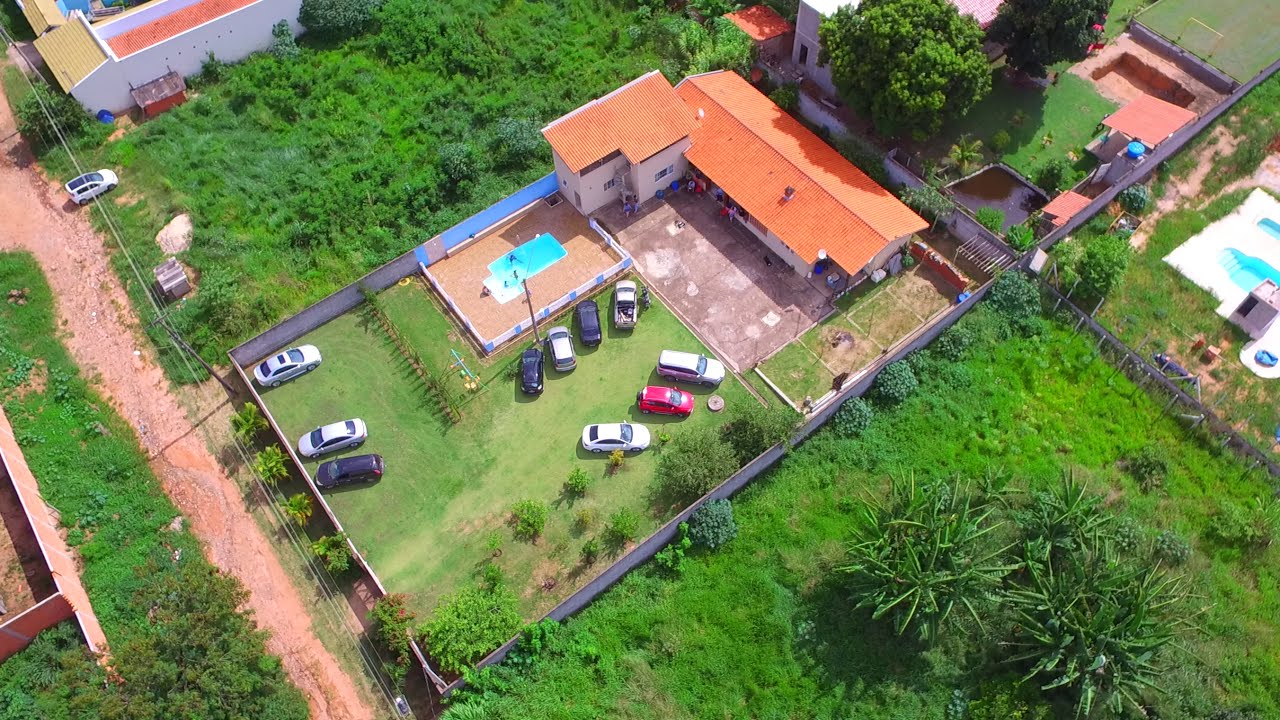This aerial photograph captures a detailed view of an outdoor scene centered around a residential area, possibly an apartment complex or hotel, characterized by its distinctive orange slated roof and off-white exterior. Enclosed by a white fence, the property features a verdant yard with lush green grass, trees, and shrubbery. Prominently situated near the back of the plot, the house is accompanied by approximately 10 cars parked at an angle in what appears to be a designated parking area. The central yard includes a small swimming pool filled with blue water, complemented by a large stone patio in the front. Surrounding this fenced area are additional patches of grass and shrubbery. Behind the main house, another building, partially obscured by large trees, is visible. To the left, another lot filled with bushes and shrubbery leads to a partially visible building. A dirt road runs behind these buildings, where a white van is parked near the partially seen structure.